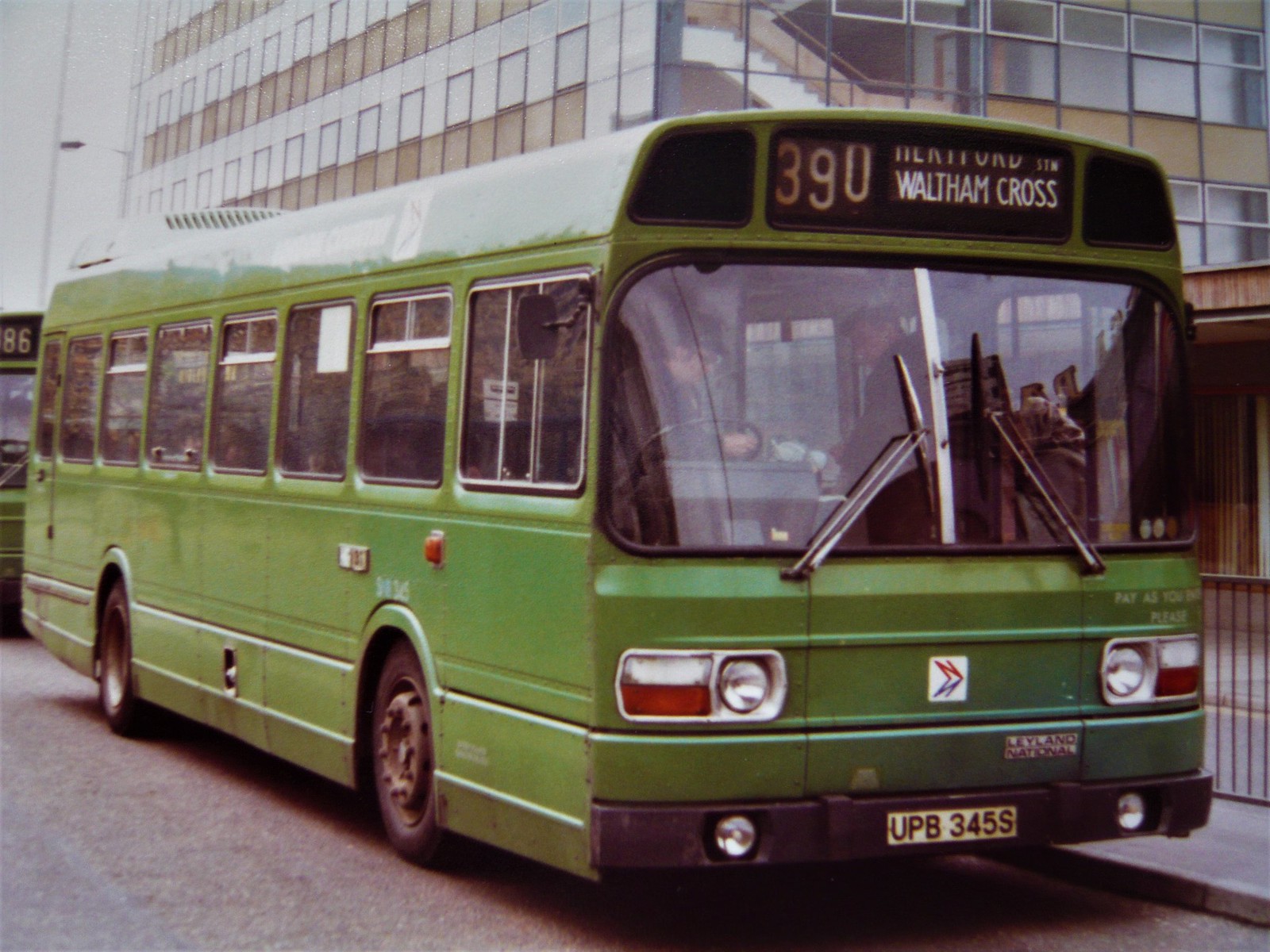In this vintage photograph taken outdoors, the setting appears to be a busy bus station in front of a large building. Two green buses are visible, with one prominently displaying the route number 390. The bus has a black sign with white lettering indicating its destination as "Walton Cross." A gate is visible on the opposite side of the bus. The design and color scheme of the buses, which are an olive green, suggest that the image dates back to the 1960s or 1970s. The buses themselves have an older, classic appearance that distinguishes them from modern city buses.